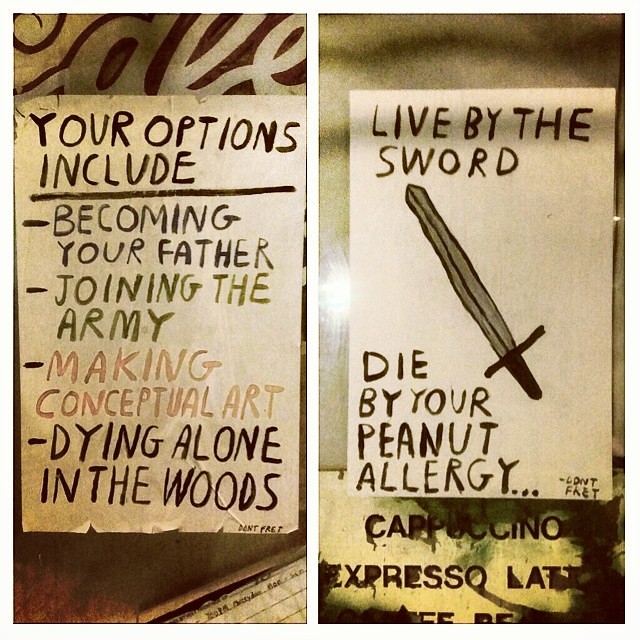The image displays two vertically split posters, side by side. On the left, a worn piece of paper with torn edges captures the eye. Handwritten text at the top reads "YOUR OPTIONS INCLUDE," followed by several life choices in a list format: "Becoming your father, Joining the army, Making conceptual art, Dying alone in the woods." Small black text at the bottom right states, "Don't fret." Behind this, a faint background with white text at the top and a form or folder in the bottom right corner completes the look.

The right poster features a predominantly white background with hand-drawn or painted text in all caps. It declares "LIVE BY THE SWORD," beside a diagonal outline of a sword in silver and black. Below, the text continues, "DIE BY YOUR PEANUT ALLERGY..." with "DON'T FRETTING" in caps at the bottom right. This poster appears to be mounted on a faded, worn sign advertising "Cappuccino, Espresso, Latte," hinting at its old, weathered nature. Both posters exhibit a sense of age and wear, likely drawn with paint or a paintbrush, adding to their intriguing and rustic appeal.